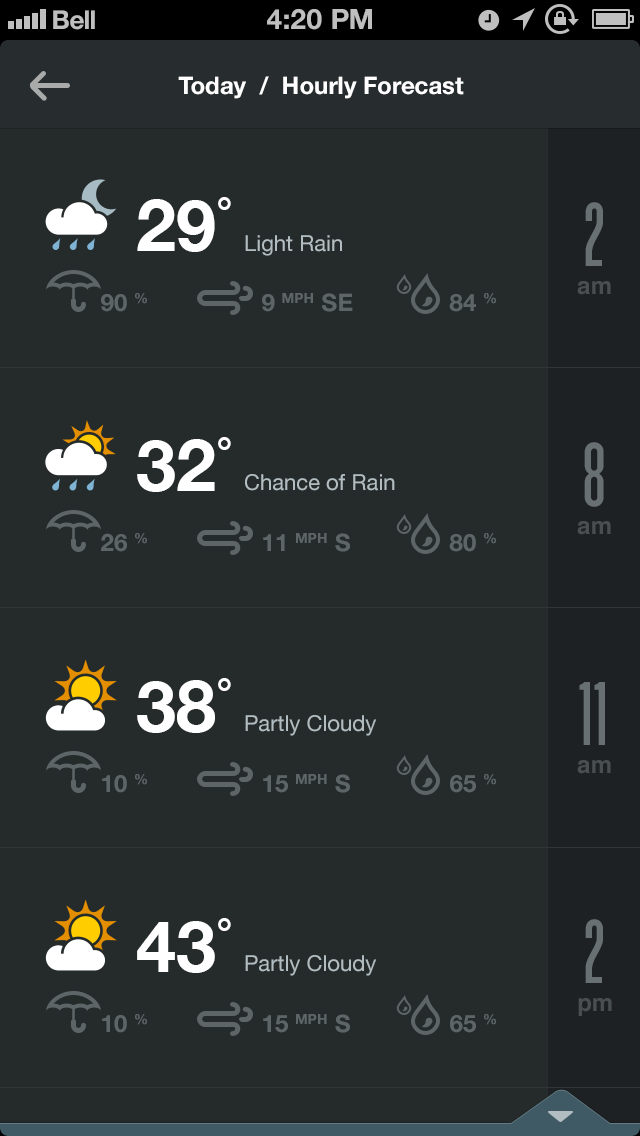The screenshot captures a weather forecast page on a mobile device, specifically an iPhone. In the top-left corner, all five bars of the network signal indicate a strong connection from the provider Bell. The screen displays the time as 4:20 PM, alongside icons for an active alarm, location services, screen rotation lock, and the battery status.

The weather page offers both current and hourly conditions. Presently, it's 29 degrees Celsius with light rain and a 90% chance of precipitation. The wind is blowing from the southeast at 9 miles per hour with a humidity level of 84%.

The forecast details for the upcoming hours are as follows:
- At 8 AM: 32 degrees Celsius, 26% chance of rain, with a south wind at 11 miles per hour and 80% humidity.
- At 11 AM: 30 degrees Celsius, partly cloudy, 10% chance of rain, with a south wind at 15 miles per hour and 65% humidity.
- At 2 PM: 43 degrees Celsius with a 10% chance of rain.
- At 4 AM: 30 degrees Celsius with a 10% chance of rain.
- At 4 PM: 30 degrees Celsius with a 10% chance of rain.